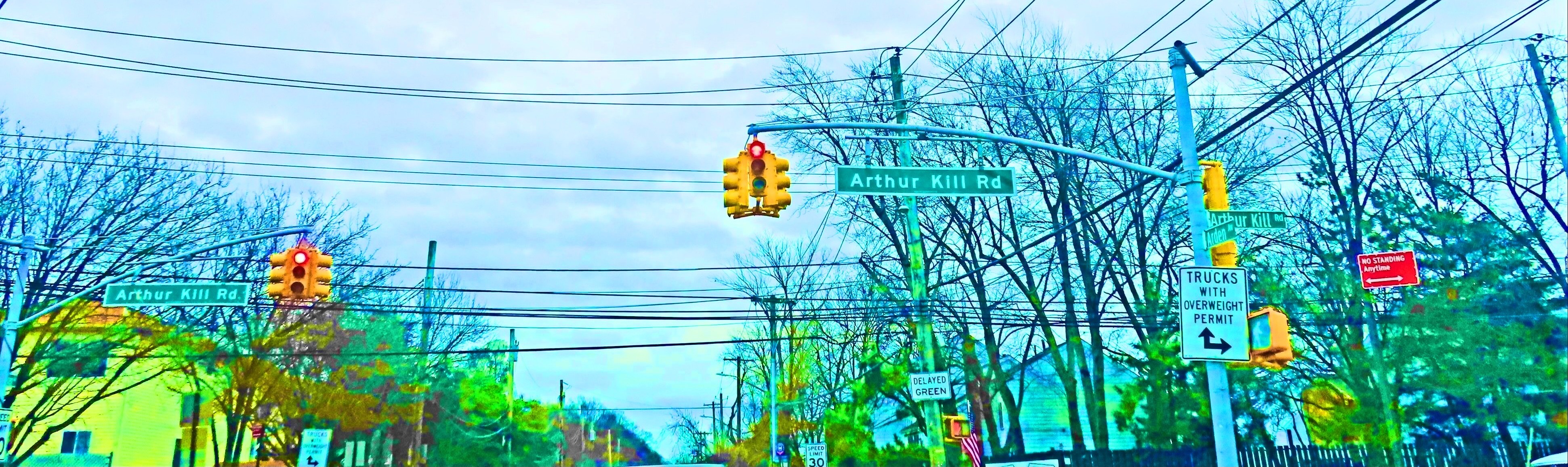This photograph has been heavily color-modified to create a cartoon-like effect with exaggerated blues, greens, and yellows. The scene appears to be a busy residential street view, likely taken from inside a vehicle, with a close-up of an intersection dominated by a four-way traffic signal. Prominently featured is a green street sign with white lettering reading "Arthur Kill Road." There are multiple yellow traffic lights, all currently red, and one additional sign with unreadable red writing. The backdrop includes numerous telephone poles and a maze of crisscrossing power lines. The blue sky and tinted foliage add to the surreal quality of the image, which also shows glimpses of houses, including one notably large yellow house on a corner, and various other rooftops. A utility sign nearby indicates directions for trucks, adding to the complexity and utility of the scene. The colors have been amplified to such an extent that the scene takes on an almost fantastical appearance.